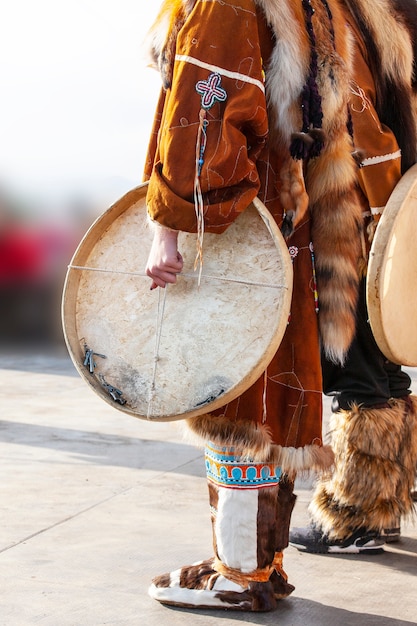In this rectangular outdoor daytime photograph, measuring approximately four inches high and three inches wide, two individuals are dressed in traditional North American Indigenous attire. Centered from the shoulders down, the person in the foreground wears a brown, long-sleeved tunic adorned with brown and cream fur trim at the bottom, and a distinctive tail featuring rings of browns, orange-browns, and creams that drapes down from their shoulder area. Their boots, crafted from white and brown fur, showcase intricate blue, orange, and red beadwork near the top. They hold a flat, circular drum-like instrument with four strings extending from its edges and meeting at the center.

The second individual stands slightly behind, wearing black pants beneath their fur-skinned leg coverings, which expose regular black and white footwear. Their black tunic and fur accents complement the attire of the person in front. This person also holds a similar round drum instrument.

Both figures face towards the left, standing on what appears to be a concrete surface. The overall color palette of their costumes is dominated by shades of brown and white, with notable blue, orange, and golden accents on the footwear and accessories. The blurred sky is visible in the upper left corner of the image, adding a soft backdrop to the rich, intricate details of their traditional attire.